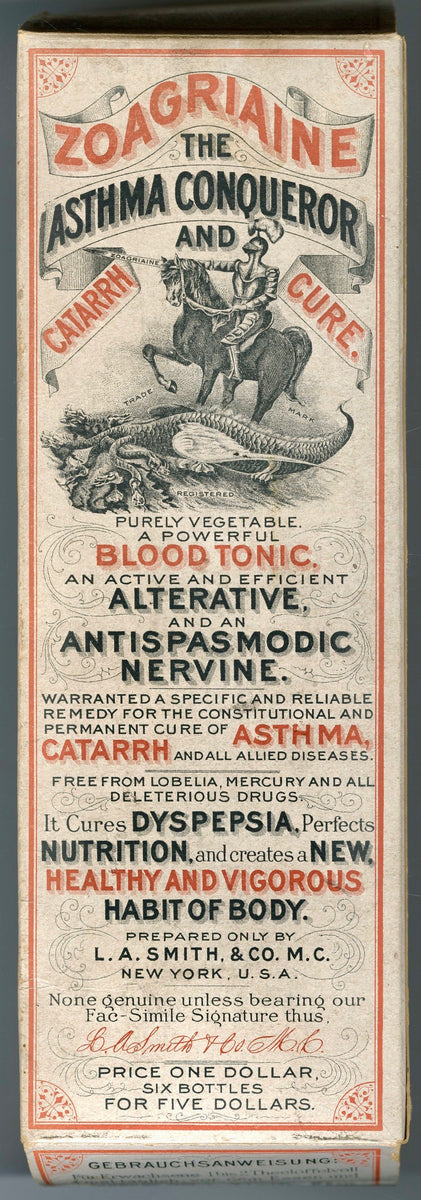The image depicts a close-up of an old, vintage advertisement on white paper, with bold red and black lettering. Dominating the top part of the ad is an illustration of a figure on a horse. The text, prominently reading "Zoa Green," announces it as "the asthma conqueror and Qatar cure." According to the description, it is a purely vegetable-based remedy boasting several benefits: a powerful blood tonic, an active and efficient alternative, and an antispasmodic. It is also touted as a reliable remedy for the constitutional and permanent cure of asthma, Qatar, and allied diseases. The advertisement highlights its safety, stating it is free from Lobelia, Mercury, and all deleterious drugs. It claims to cure dyspepsia, enhance nutrition, and foster a new, healthy, and vigorous habit of body. The product is prepared exclusively by L.A. Smith & Co., M.C., New York, U.S.A. The bottom of the advertisement notes the price as $1, or six bottles for $5. The visually striking ad, with its antique charm, presents text in multiple languages, with some portions in French, and emphasizes the authenticity of the product with the company's facsimile signature, all set against a tan background with reddish-orange and gray printing.